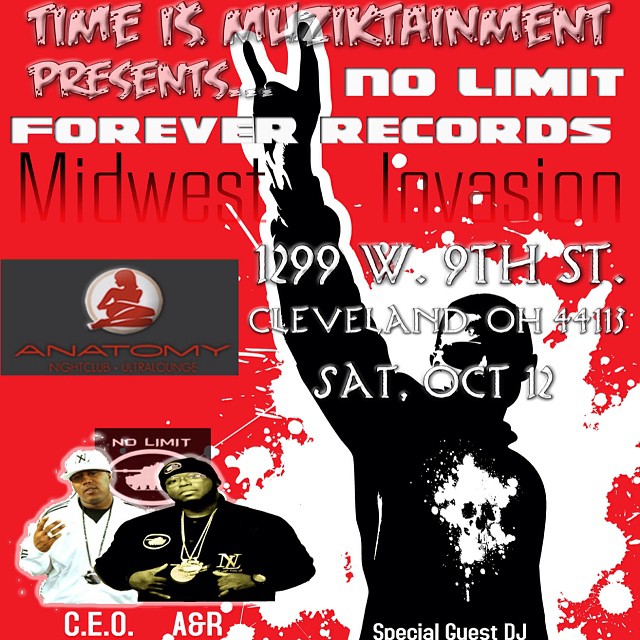This promotional flyer for the music group features a prominent red and white background, and announces "Musictainment presents No Limit Forever Records Midwest Invasion," taking place at the Anatomy Nightclub Ultra Lounge, located at 1299 West 9th Street, Cleveland, Ohio, 44113, on Saturday, October 12th (no year provided). The design includes an image of two black men at the bottom left, one dressed in all black and the other in all white, both wearing chains and hats – one in a cap and the other in a beanie. Identified as CEO and A&R respectively, they're shown displaying different hand symbols. Additionally, there's another image of a man in a black t-shirt with a skull graphic, throwing up the rocker sign. The poster's color scheme includes red, white, black, pink, brown, and tan, with most of the text positioned at the top and right side of the image. This flyer is a vivid, eye-catching advertisement for an upcoming event at the nightclub.